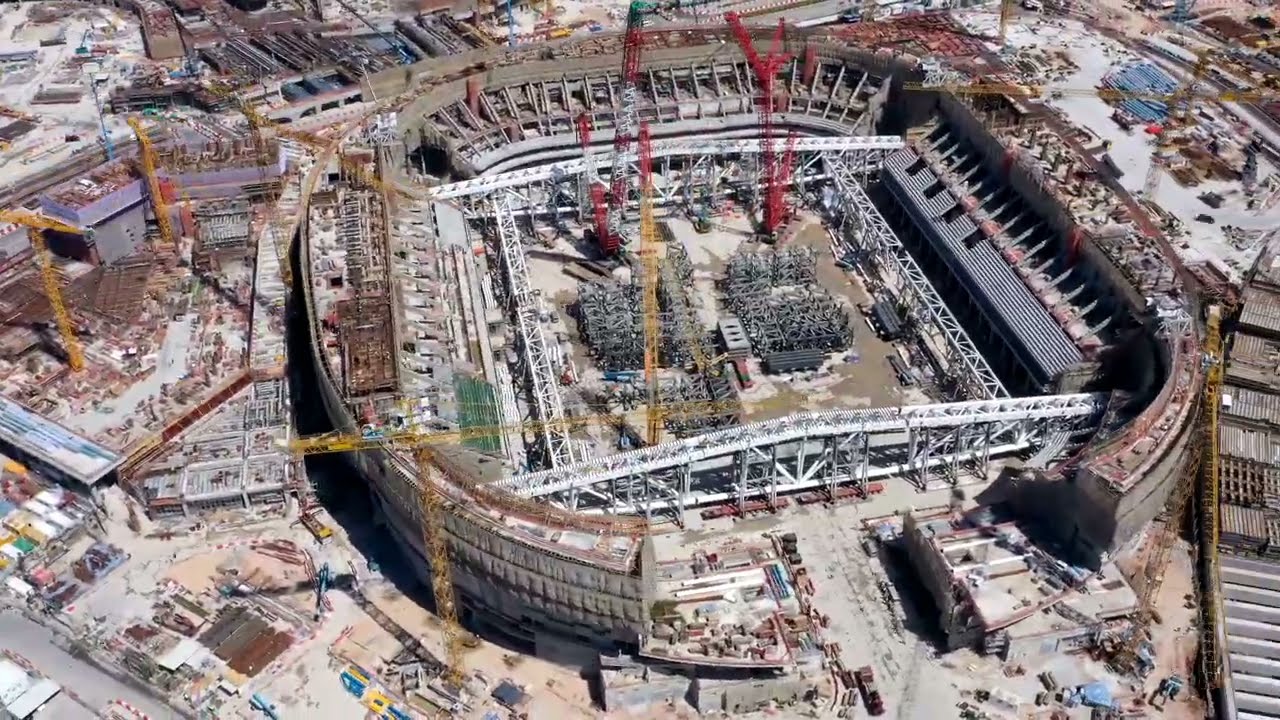The overhead photograph captures the extensive construction of an outdoor stadium or arena, possibly a colosseum or concert hall. The image reveals a partially built structure with completed sections on the right, left, and back sides, while the front portion remains unfinished. Inside the stadium, rows of green and gray seats are visible amidst extensive metal scaffolding.

Dominating the construction site are several large cranes: a massive yellow crane at the front, a bright yellow crane in the middle, a striking bright red crane behind it, and a red and white striped crane to the left. Additional yellow cranes are positioned outside the stadium. The stadium itself largely appears gray and white due to its incomplete state, with isolated sections exhibiting these colors.

Surrounding the stadium, the landscape is bustling with construction activity, including trucks, cars, and building supplies. The ground outside looks snowy white, suggesting recent snowfall and emphasizing the construction's scale and intensity. Across both ends of the stadium are silver brackets or beams adding to the complex structure. Additionally, the wider area features ongoing development with new buildings, parking lots, and stores being constructed, signaling a comprehensive transformation of the entire vicinity.